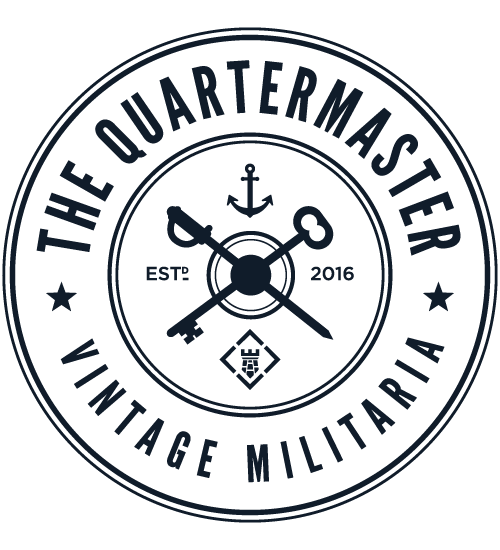The logo is a black and white circular insignia composed of two concentric circles, bordered by a thin and a thick black line with a white line in between. In large, black capital letters, it reads "THE QUARTERMASTER" at the top and "VINTAGE MILITARIA" at the bottom along the perimeter. Flanking the sides are two stars. Central to the design is a coat of arms featuring a sword and a key crossed, dividing the circle into four quadrants: the top quadrant contains an anchor, the right quadrant shows the year "2016," the bottom quadrant displays a diamond with a rook or castle inside it, and the left quadrant bears the abbreviation "EST" followed by a smaller "D." The overall impression is reminiscent of a tire, with detailed elements in the middle akin to a hubcap.